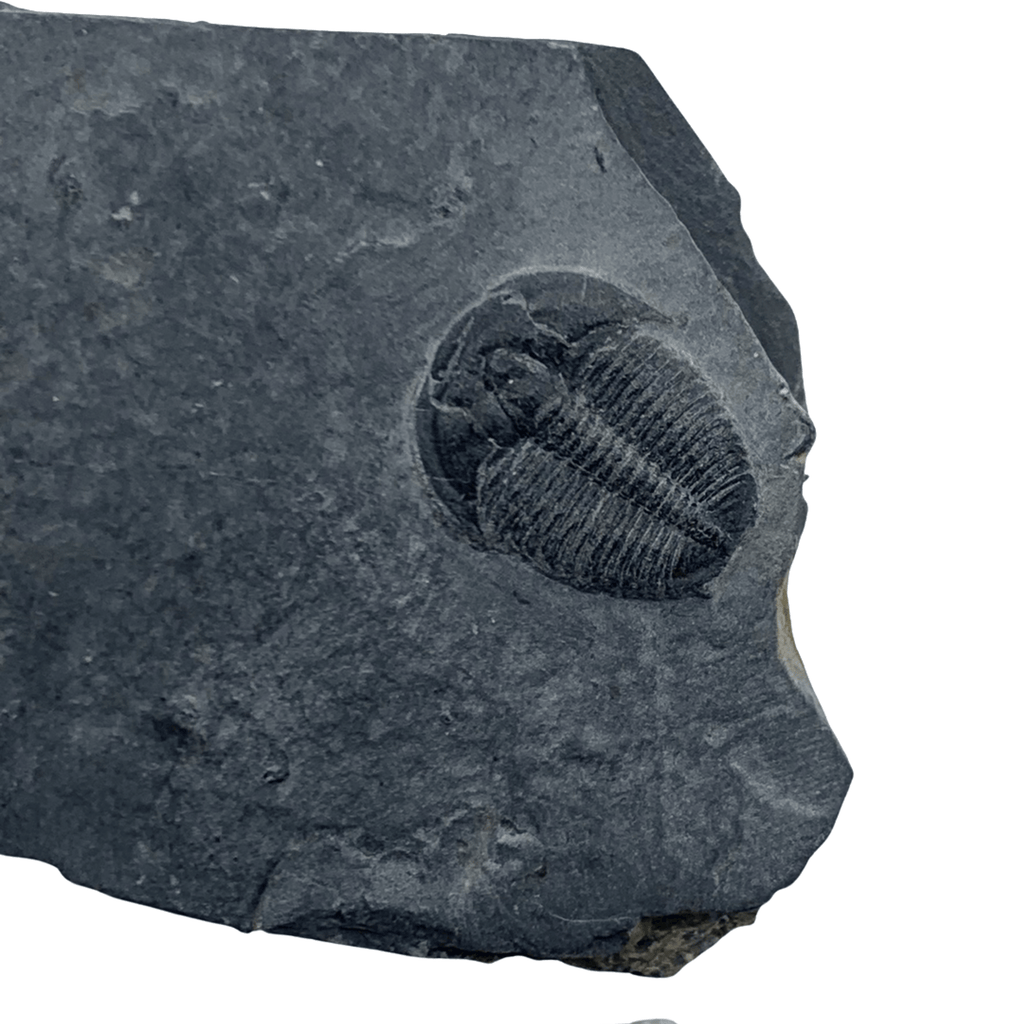This highly detailed photograph features a large, jagged gray rock prominently placed against a white background, primarily oriented on the left-hand side of the frame. The rock’s silhouette is reminiscent of the right side of Pennsylvania’s border, with a nearly vertical left edge and a smoother, almost horizontal top. On the right side of the rock, in the upper portion, there is a fossil embedded, angled at approximately 45 degrees. The fossil, possibly of a crustacean or insect, displays intricate characteristics: the lower section showcases vertical lines running across it, while the upper section forms a semicircle featuring a central raised bump. The fossil blends seamlessly within the gray hues of the rock, yet remains striking due to its detailed preserved patterns, evoking a sense of ancient life encapsulated within the stone. Some interpret the rock's shape as resembling an animal's head, with fossilized markings suggesting features like an eye and a snout. This captivating geological and paleontological specimen connects the viewer to millions of years of Earth's history, preserved in stone.